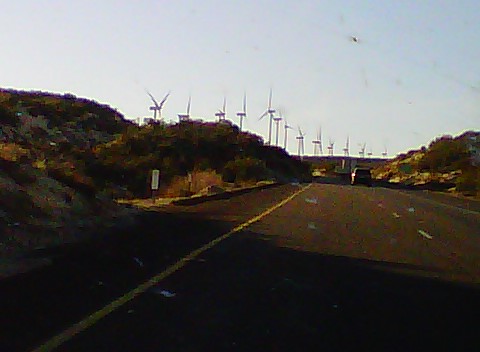This color snapshot captures a desolate, hilly landscape dominated by a long, two-lane road stretching into the distance. Flanking both sides of the road, there's sparse, desert vegetation, featuring patches of green bushes interspersed with areas of dead grass. The scene is set on a series of hills, where the road navigates through an undulating terrain, marked by a dotted white line indicating passing zones. 

In the distance, over ten modern wind turbines – specifically 14 to the left side of the highway – punctuate the horizon, their sleek blades calmly rotating. These turbines are situated behind the hills, contributing to a sense of depth. The wind farm extends along a considerable portion of the backdrop, suggesting a significant investment in renewable energy in this area. 

Further along the road, there appears to be an overpass partially obscured by the distance. The pale blue sky above hints at a setting sun, indicated by the long shadows stretching across the scene. A barely discernible mile marker sign rests on the left, counting down the distance in this secluded, windy stretch.